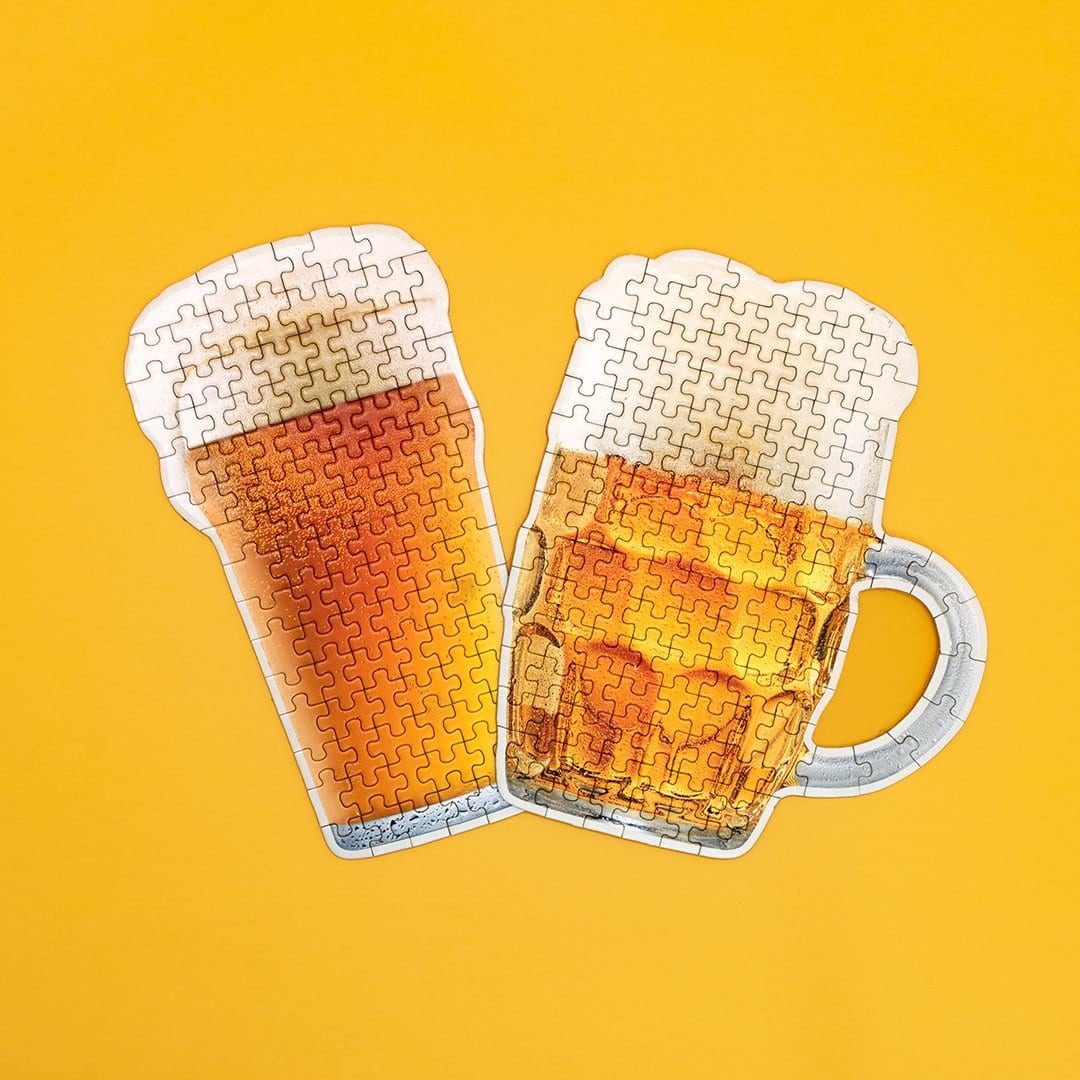The image depicts a completed puzzle against a vibrant, deep yellow background. The puzzle features two beer containers: a tall glass and a mug. Both beverages have a thick, frothy layer of foam at the top. The tall glass on the left, slightly tilted to the upper left, displays an amber-golden beer without a handle. The mug on the right, slightly tilted to the upper right, has a noticeable handle and a textured surface resembling thumbprints. The body of both the glass and the mug, including the foam and the handle, are composed of interlocking puzzle pieces. The detailed portrayal emphasizes the distinct amber-golden hue of the beer and the silvery color of the mug's handle, set against the striking mustard-yellow background.